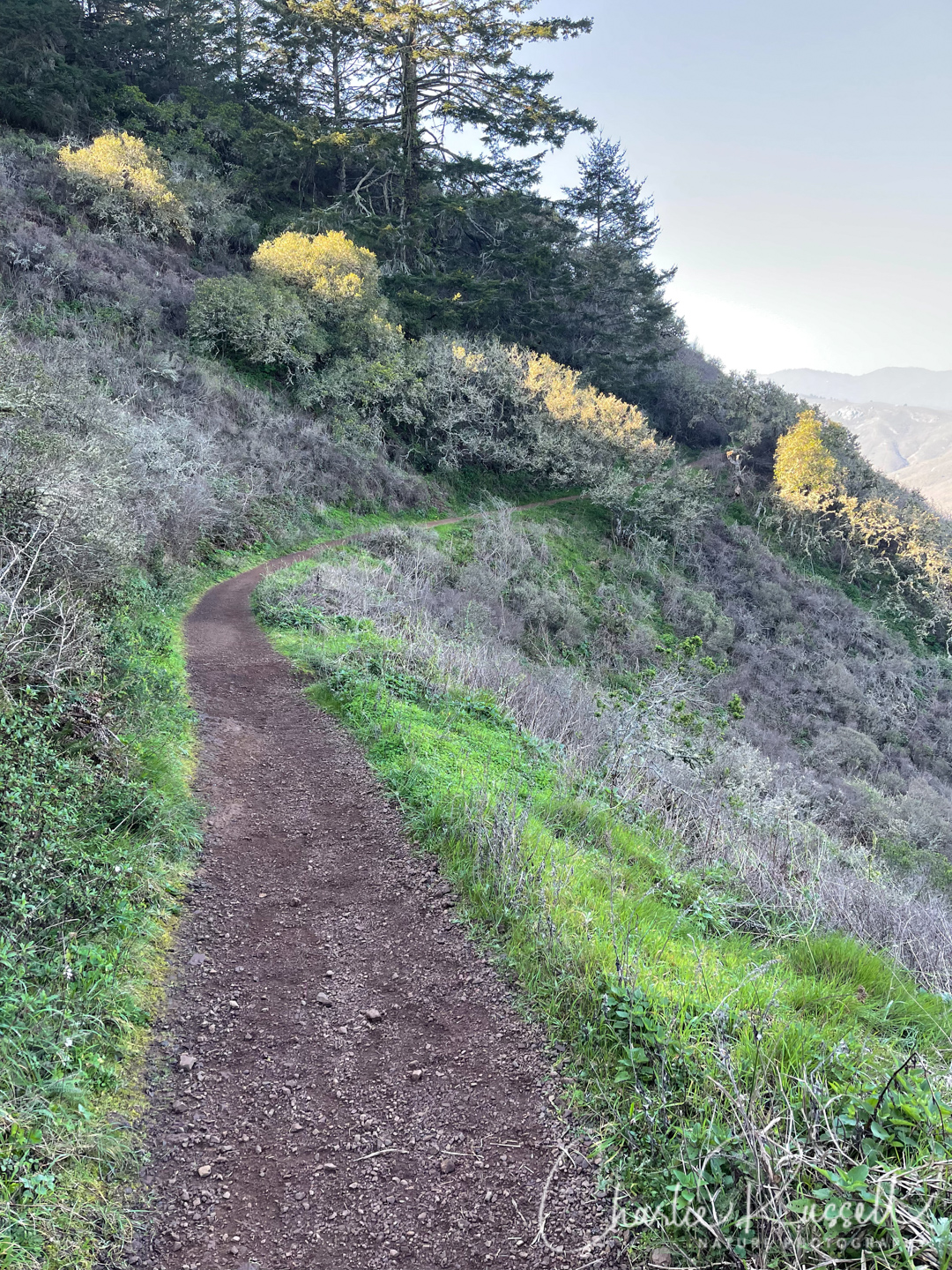The photograph, taken in portrait orientation, beautifully captures a serene hiking scene on a steep hillside. The focal point is a narrow, pebbly dirt path winding its way through the landscape, which appears suitable only for walking. The path is flanked by varying shades of green foliage, with patches of variegated green grass immediately adjacent to the walkway, transitioning to grayish-brown grass and lighter golden shrubs further out. In the upper portion of the image, dark green pine trees with dense branches and lighter colored shrubs are visible. The terrain slopes steeply from the top left of the image to the middle right, with the hill rising on the left and descending on the right. In the distance, the outline of mountains can be seen against a light blue, possibly muted, sky. A hint of sunlight suggests it could be either a cloudy day or approaching sunset. The name "Charlie Russell" is faintly discernible in the lower right corner of the image, indicating the artist's signature.